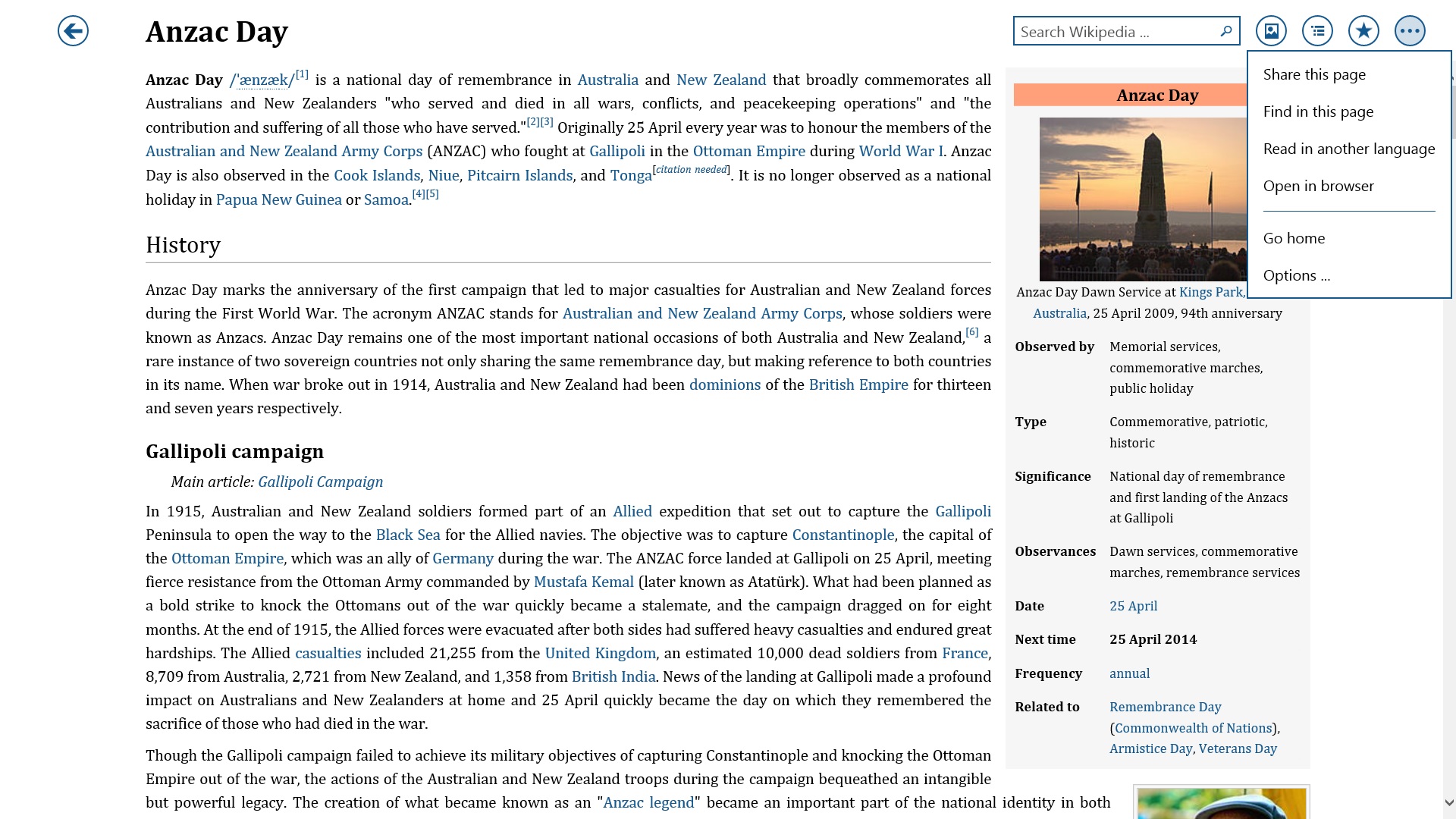"Screenshot of a mobile device showing the Wikipedia search page for 'Anzac Day'. At the top left, an arrow icon is visible, likely representing the back button. The main menu includes several options: 'Share this page', 'Find on this page', 'Read in another language', 'Open in browser', 'Go home', 'Options', a star icon for bookmarking, a circular icon, and an ellipsis for more options. The search query 'Anzac Day' is prominently displayed."